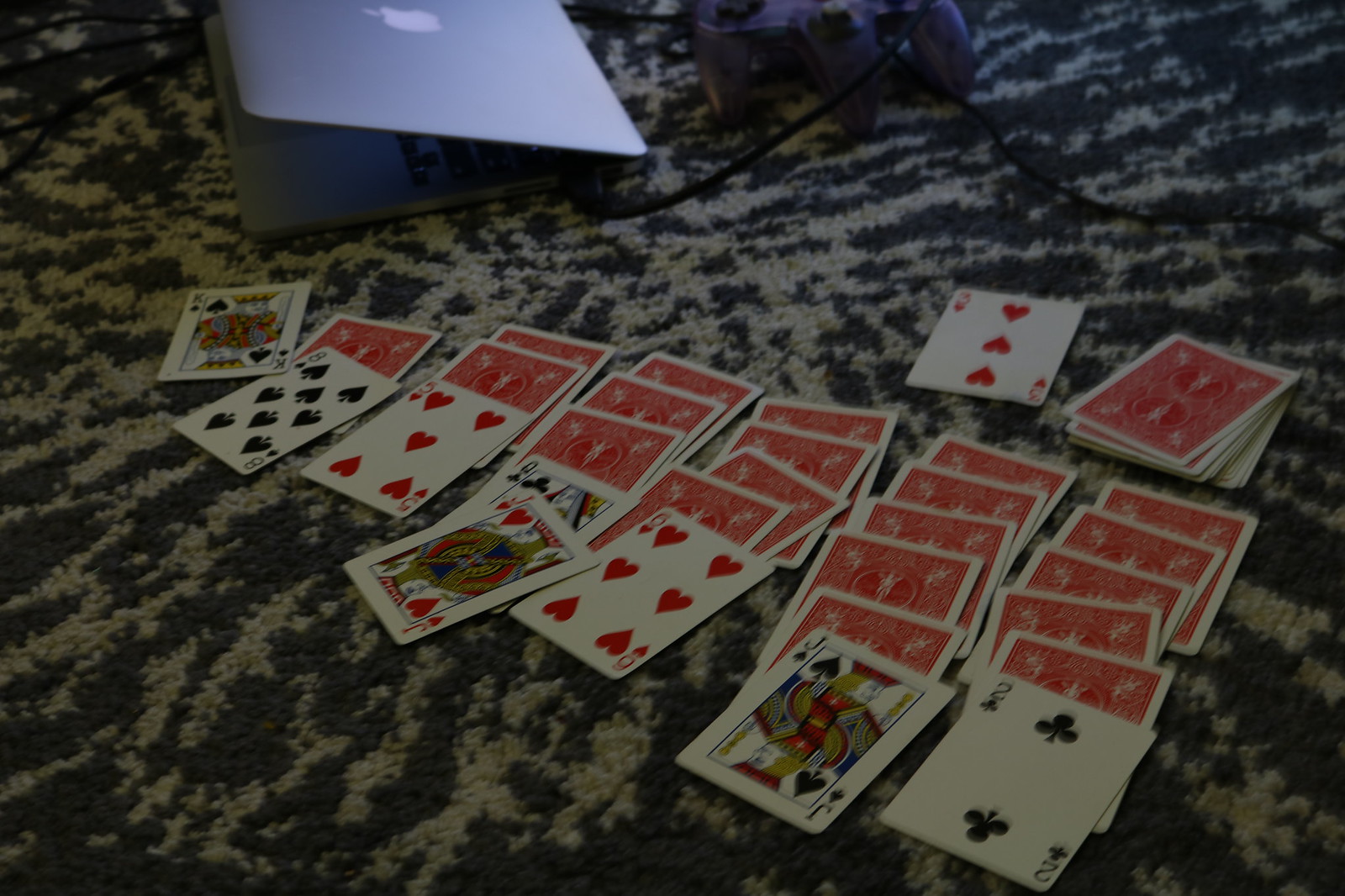A neatly arranged game of solitaire is laid out over a dual-colored carpet, featuring a staggered pattern of light, almost white, and bluish-black hues. The deck of cards is positioned towards the bottom half of the image with most of the cards facing down except for one card next to the deck and the cards at the bottom of seven rows. From left to right, the face-up cards are the King of Spades, Eight of Spades, Five of Hearts, Jack of Hearts, Queen of Clubs, Six of Hearts, Jack of Spades, and Two of Clubs. Above the card layout, additional carpeting is visible. Further up, a purple game controller with two controls and a connecting wire is discernible. To the left of the controller, a partly closed MacBook is evident, with three wires extending from its side towards the upper left corner.